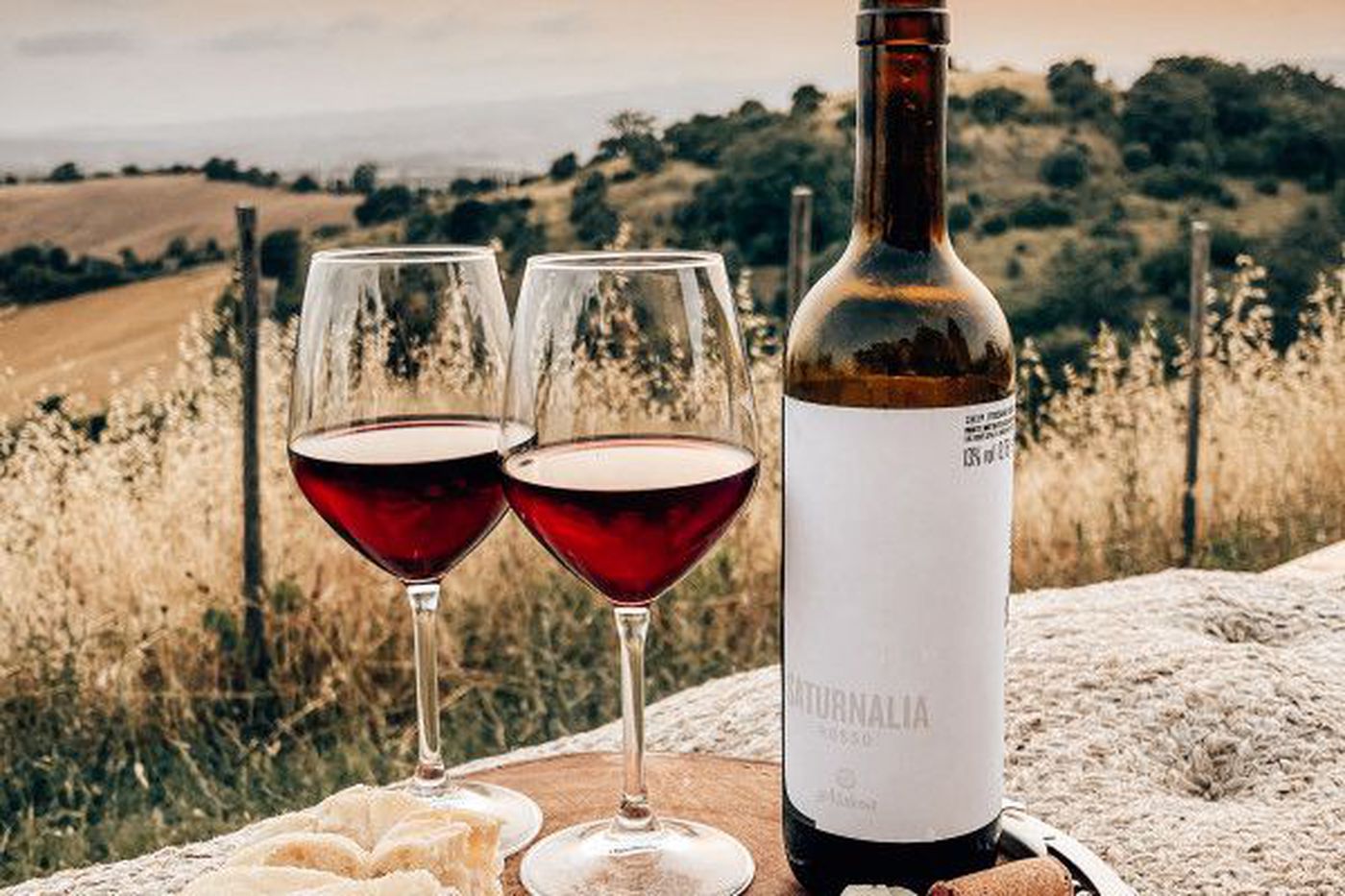This professionally done color photograph, likely used for an advertisement, showcases a picturesque outdoor setting. Central to the composition are two elegant wine glasses, a third filled with red wine, positioned side-by-side. The glasses have a slender, narrow base that widens at the bowl before tapering to the top opening. To their right is a brown glass wine bottle, adorned with a mostly blank white label containing the faded word "Saturnalia" and the numbers "530" in light and dark letters.

The scene is set atop an orange fabric cloth, which rests on an indistinct, irregular surface that appears to be a white tan sack. In front of the wine glasses, pieces of bread and a cork are visible on the cloth. The background features a stunning landscape of rolling hills with tan, wheat-like fields interspersed with clusters of plush green trees. A wired fence can be seen near the glasses, and tall yellow grass is prominently featured in the foreground. The photograph is taken during daytime under clear skies, adding to the serene and inviting atmosphere.